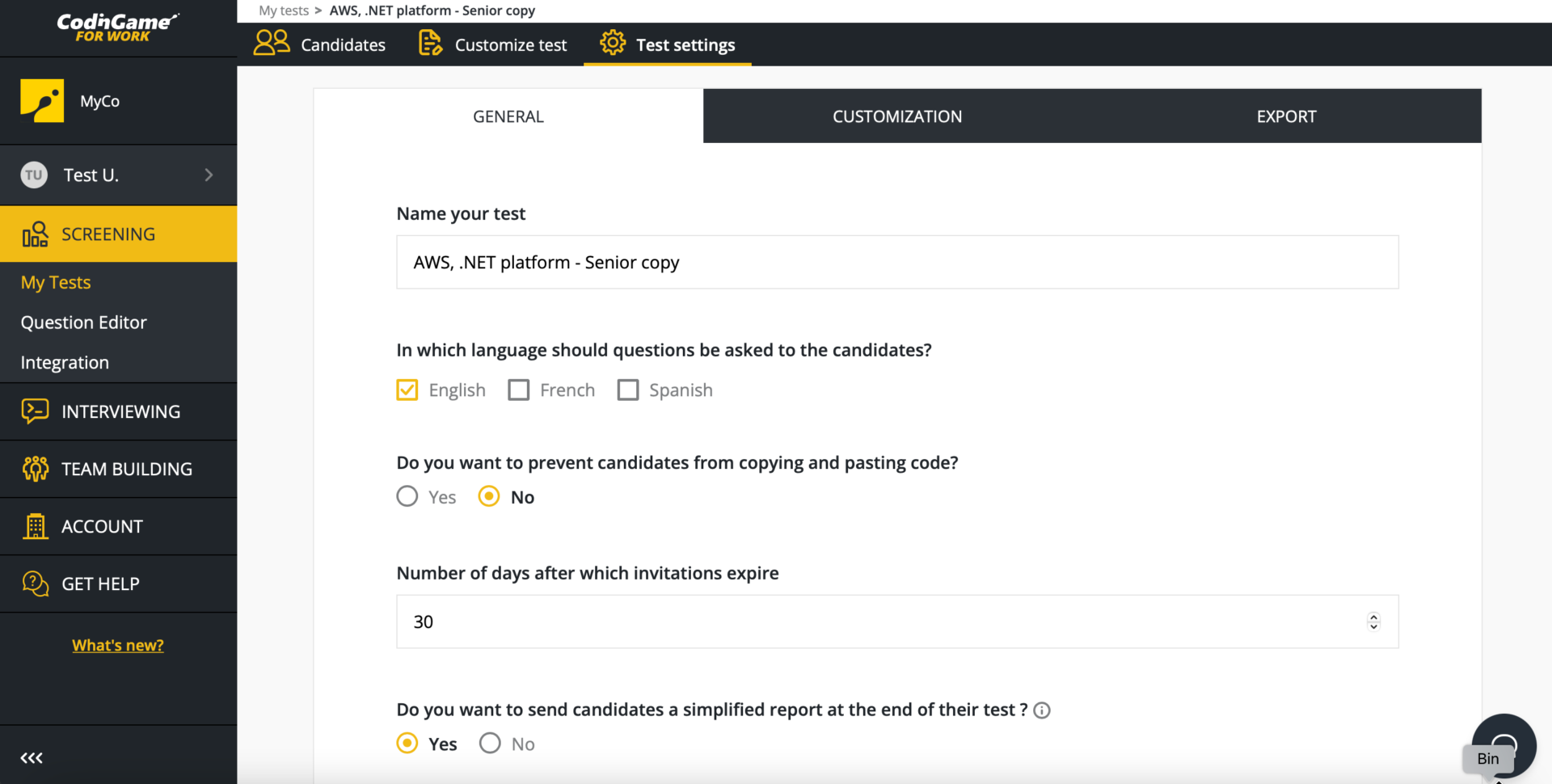Here is a detailed, cleaned-up caption for the image:

---

The image is a screenshot of a website designed for code testing. The top-left corner prominently displays the title "Coding Game for Work." On the right side of the header, text reads "Candidates Customize Text and Testing." Below this section, there are multiple options and fields for configuring a coding test. These options include "Naming Your Test," "In Which Language Should Questions Be Asked to the Candidates?", "Do You Want to Prevent Candidates from Copying and Pasting Code?", "Number of Days After Which Invitations Expire," and "Do You Want to Send Candidates a Simplified Report at the End of Their Test?"

---

This caption provides a clear, detailed description of the content and layout of the website screenshot.